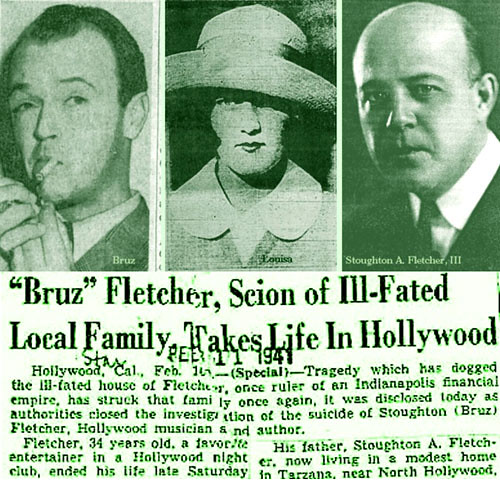The detailed caption for the image described can be written as follows:

"An old black-and-white newspaper article titled 'Bruce Fletcher, Scion of Ill-Fated Local Family, Takes Life in Hollywood,' captures the tragic end of a once-prominent family. At the top of the page, three photographs are displayed: on the left, a man with a receding hairline is seen lighting a cigarette; in the center, a woman wearing a hat, her right eye clearly visible and staring directly at the camera while her left eye is almost obscured; and on the right, an older balding man in a shirt and tie looks into the camera. Below the photos, the headline narrates the misfortune of the Fletcher family, who were once rulers of an Indianapolis financial empire. The article reveals that Stoughton Brez Fletcher, a 34-year-old Hollywood musician and author, ended his life on Saturday in Tarzana, near Hollywood. The family, once entertainers in Hollywood, now lived modestly, marking another chapter of tragedy for the ill-fated house of Fletcher."